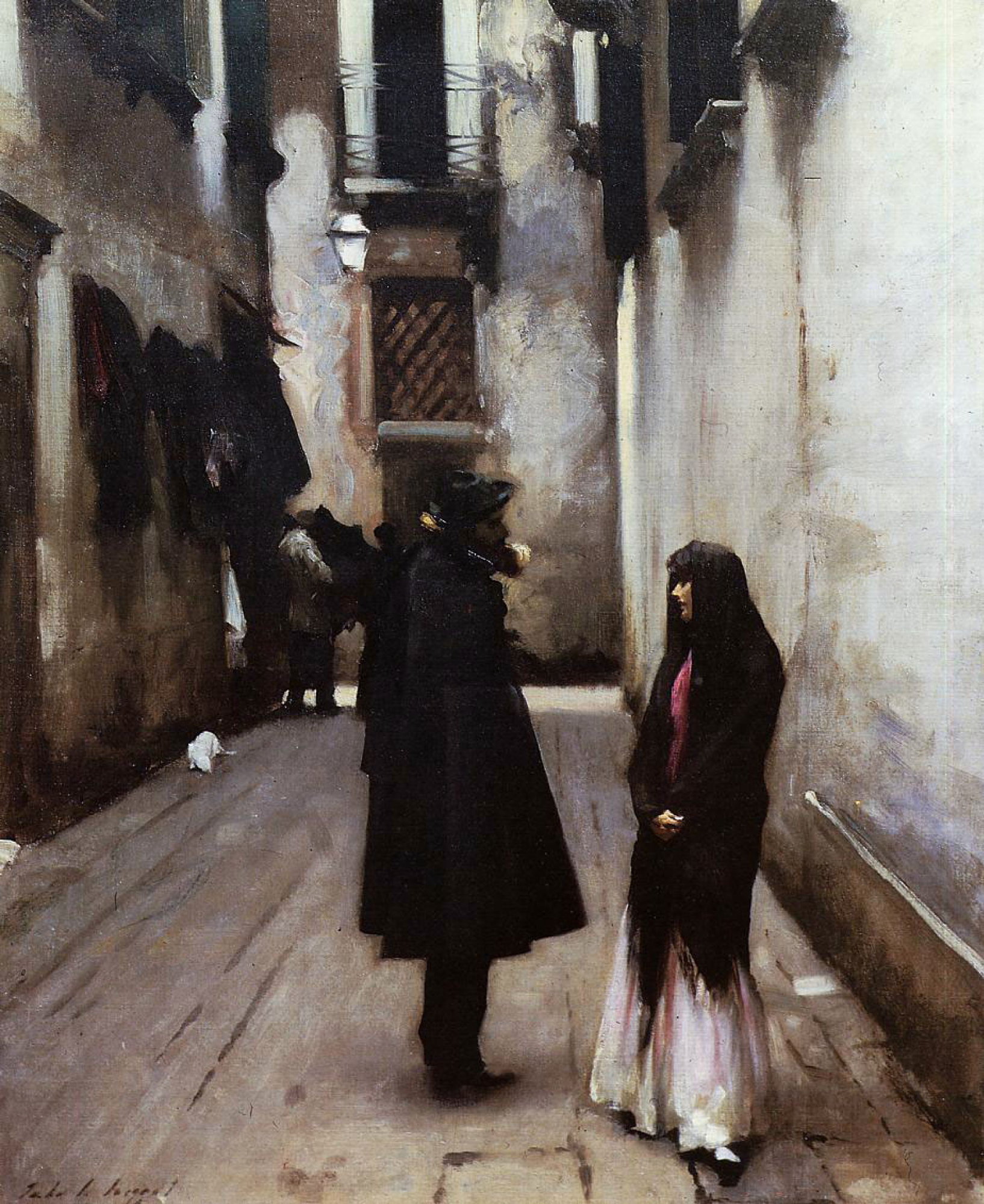In this dreary, abstract alleyway painting characterized by muted grays, blacks, and pale pinks, two figures dominate the foreground with a striking presence. To the left stands a man dressed in a black hat, black trench coat, and matching dark shoes. His face is obscured by an indecipherable mask, lending an air of mystery. Opposite him, a woman clad in a black and pink gown, complete with a dark veil and shawl, crosses her hands as she gazes at the man. Her dress extends graciously to her ankles, highlighted with subtle pastel pinks. White walls bracket the figures, punctuated by windows and lights that dimly illuminate the scene, while the wooden floor underfoot suggests an interior space. Near the base of the wall on the left, a small creature — possibly a mouse or a cat — subtly blends into the subdued palette.